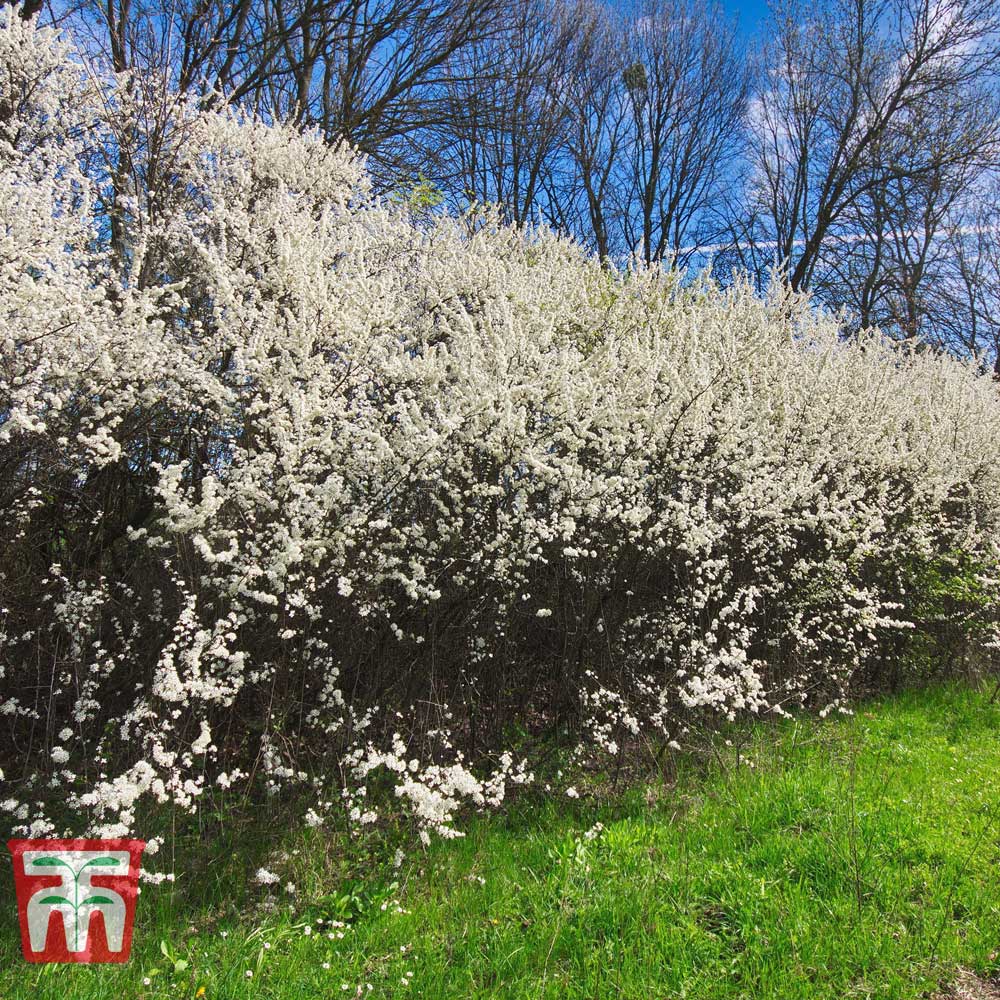This square photo captures an outdoor scene in a garden or yard, showcasing a vibrant display of nature. The foreground features a sprawling area of bright lime-green grass, which is uneven in height, interspersed with wild grasses and possibly some weeds. Dominating the middle of the frame, a large bush stretches across from left to right, densely covered with small, delicate white flowers that resemble popcorn or cotton from a distance. The bushes have dark brown, thin branches visible through the blossoms, adding to the scene's intricate texture. 

In the background, leafless trees with dark, sprawling branches point in various directions, hinting at an early spring setting before the buds have fully emerged. Above the trees, a vivid blue sky with fluffy white clouds completes the bright and sunny atmosphere. The bottom left corner of the image contains a distinctive red shape with white and green markings, possibly a logo. The blend of natural elements and the clear, distinctive sky create a lively and refreshing outdoor snapshot.